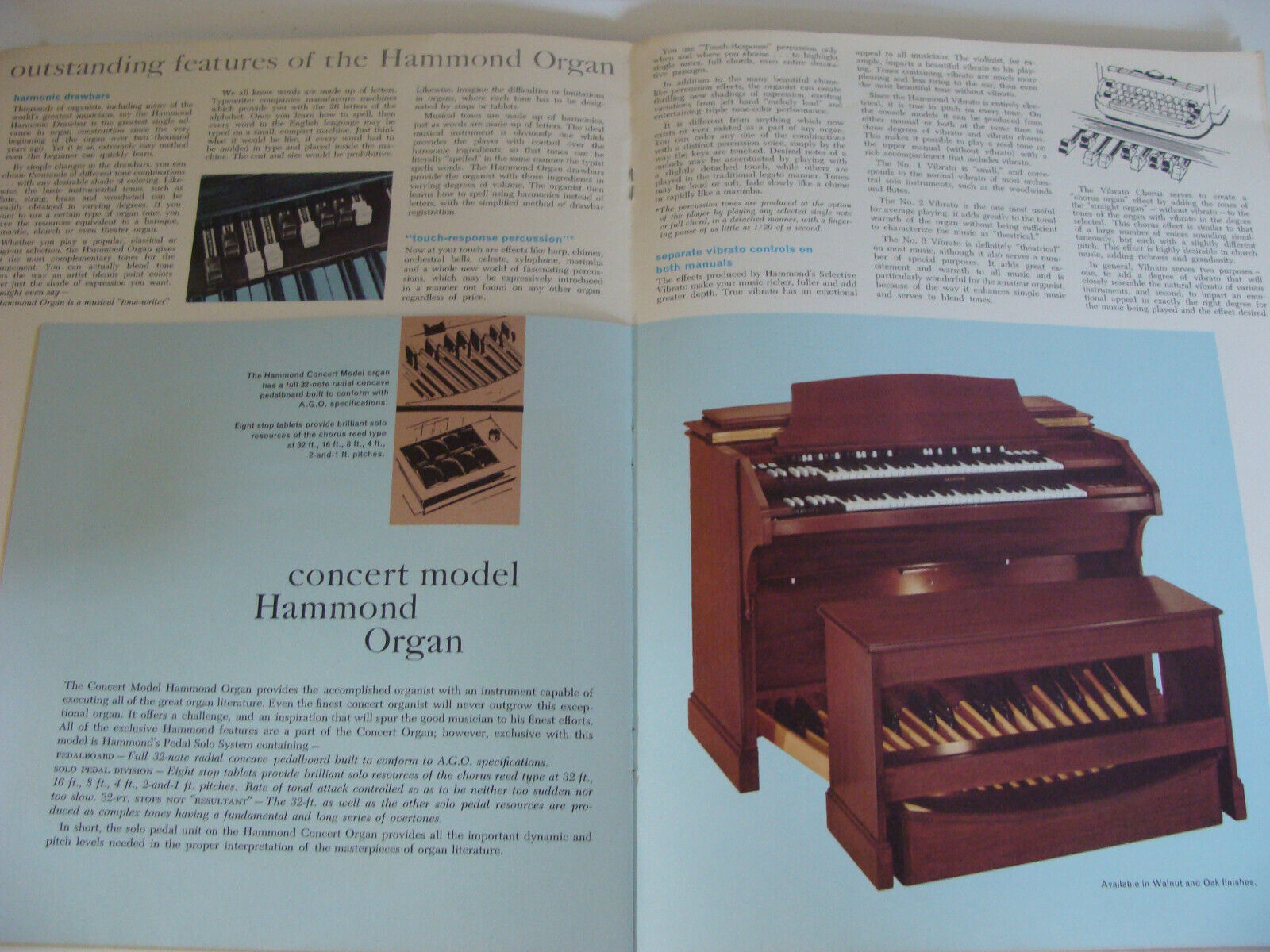This image appears to be a detailed spread from a magazine or book, showcasing the outstanding features of the Hammond organ. The top left corner displays the text "Outstanding Features of the Hammond Organ" against a white background. The centerpiece of the layout is a section with a blue background, prominently featuring a large wooden organ, finished in a cherry-looking wood. The organ is described as a concert model and is equipped with numerous keys arranged in two rows, along with many foot pedals. To the right of this section, there's an illustration of the organ in black and white, providing a detailed view of its keys and possibly some internal components or pedal diagrams. 

The layout includes an area for sheet music on the organ, and a long bench for the player. Additional text on the left side of the image reiterates the "concert model Hammond organ," accompanied by more small print details, which are too small to read clearly in the image. The overall presentation, complete with multiple columns and sections, suggests it is an informative piece meant to highlight the various features and specifications of the Hammond organ, likely intended for enthusiasts or potential buyers.